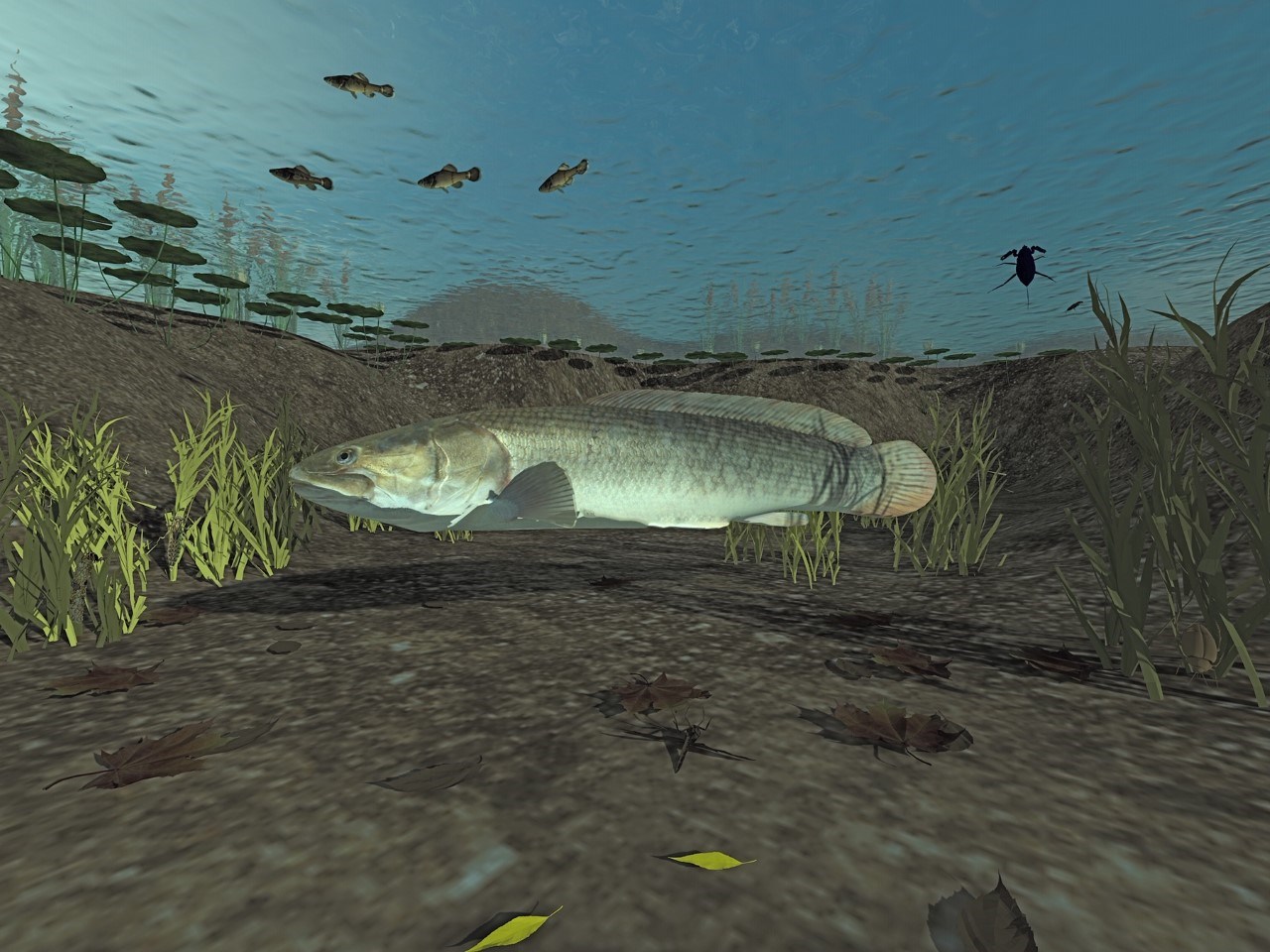An underwater, 3D CG image showcases a silvery, long fish resembling a bass as the central focus. The fish is situated near the pond or lake bottom, surrounded by seaweed or kelp growing from the brown, indented floor. Above, the water's surface reveals a blue sky and floating lily pads. Four smaller fish are visible close to the surface, accompanied by a silhouetted water bug on the right-hand side. Reeds and a possible mountain in the background complete the scene. The image, with its basic, old computer game graphics, provides a detailed underwater perspective.